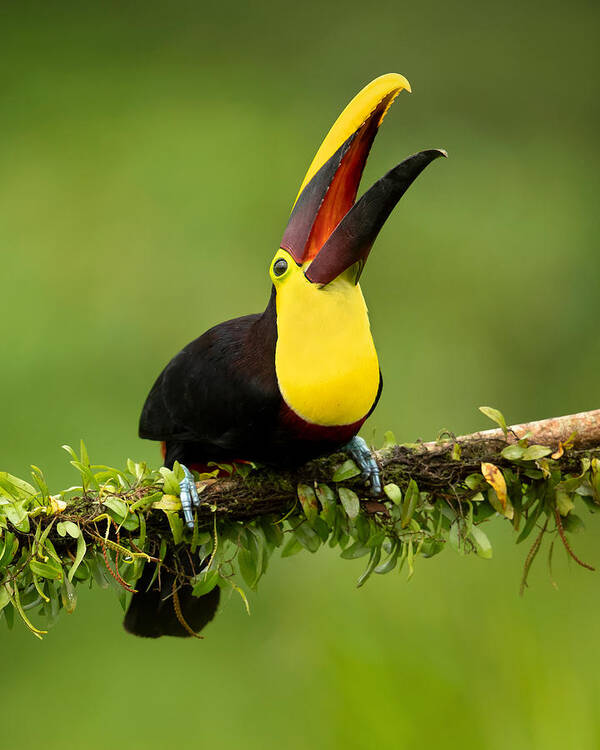The image showcases a striking scene of a toucan perched on a branch that stretches across the middle of the frame. The branch is enveloped by vines and leaves, particularly concentrated on the left-hand side. The toucan, with its dark silky black body and vibrant yellow neck, stands out as the central focus. It sits with its feet grasping the branch, its wings visible, and its head tilted upwards with its mouth open, revealing a red interior. The beak is a distinctive mix of colors: the top part is a vivid yellow while the lower part is black with hints of red. Only the right side of the toucan is visible, including its black eye. The background is a blurred green, creating a serene, natural outdoor setting where the branch and the bird remain in sharp focus. This detailed composition captures the essence of nature with the bird seemingly caught in an action, possibly singing or calling out.